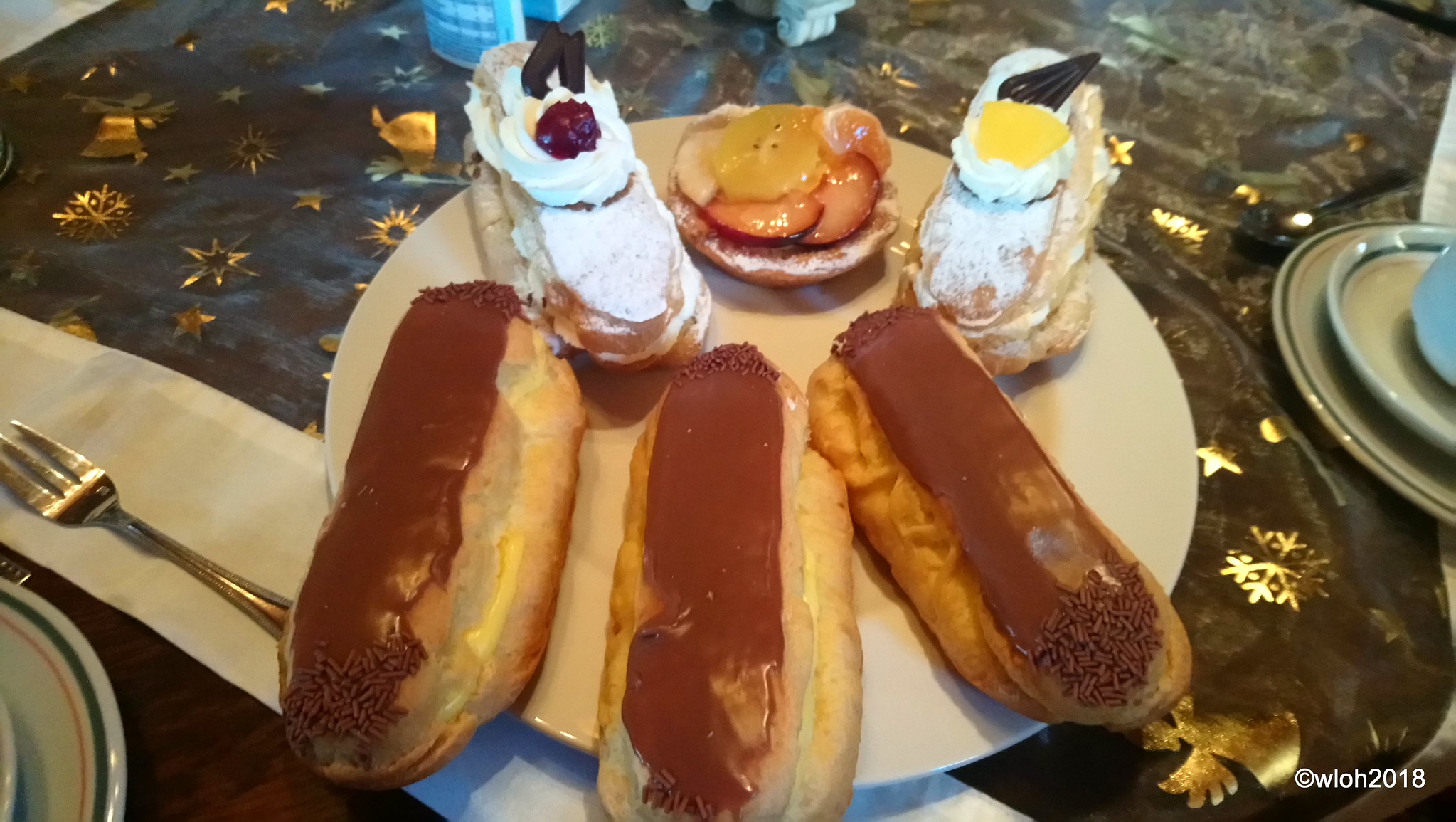This color photograph showcases an assorted array of intricately decorated pastries presented on a beige plate. Dominating the arrangement are three chocolate eclairs, their glossy chocolate frosting adorned with colorful sprinkles. There's also a smaller round pastry featuring a golden brown glaze and topped with a decorative stamp bearing "WLOH 2018." Beside these eclairs, the plate also holds two pastries that could be cannolis, each crowned with different toppings: one with a bright yellow lemon-like garnish and the other with what might be a blackberry or a maraschino cherry. Complementing the scene, the plate is set against an elegant tablecloth with golden accents, perhaps suggesting a festive or holiday theme. Near the plate, a neatly folded napkin and a silver three-pronged fork are arranged, while a stack of two plates with a mug atop can be seen in the background.